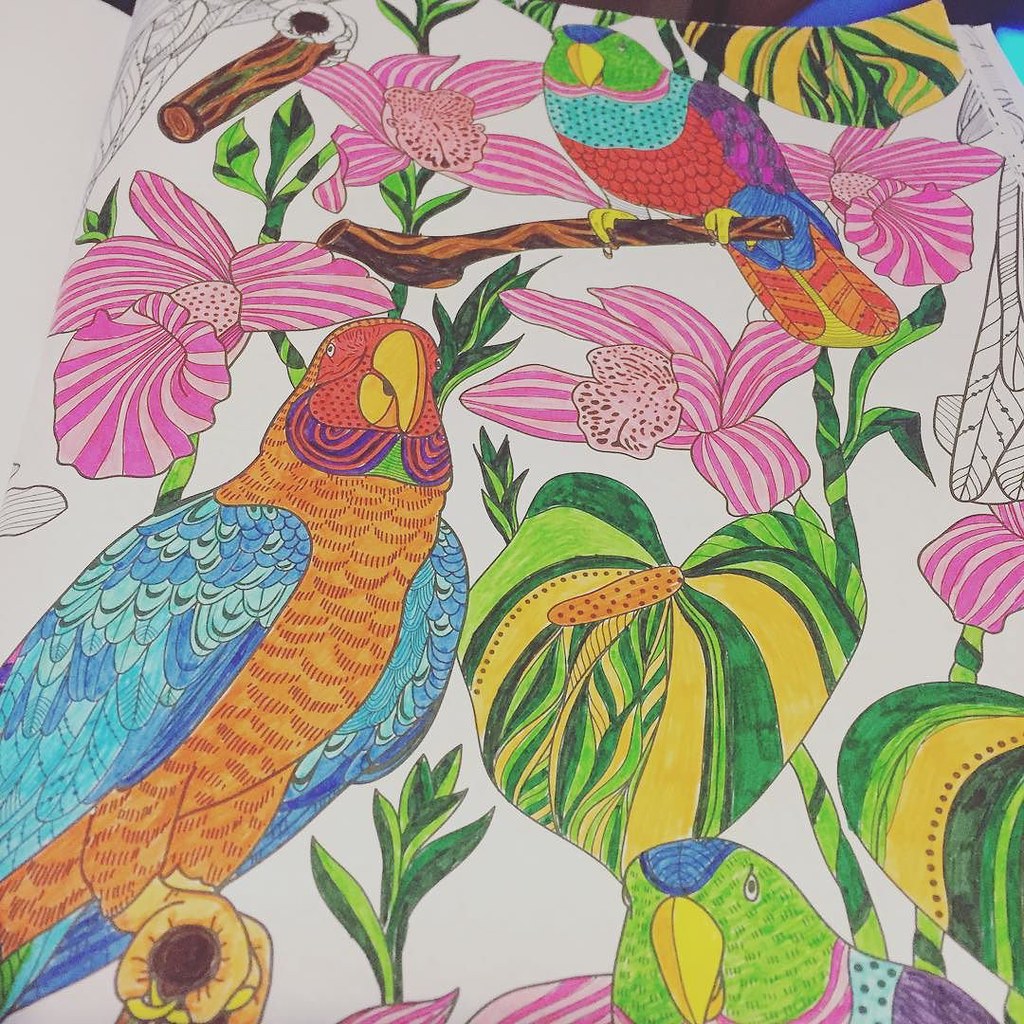The image showcases an intricately drawn and vividly colored artwork, potentially executed on fabric, featuring an array of birds, flowers, and lush foliage. The lower portion of the image prominently displays three birds, each distinctively detailed. Positioned centrally at the bottom, only the head of a bird is visible, gazing directly forward with keen eyes. To the left of this bird, another bird can be observed, displaying striking blue feathers complemented by an orange body and a vibrant yellow beak. Above this bird, perched gracefully on a sturdy brown branch, is a third bird. This bird captivates the viewer with a red and aqua blue torso, a green head, and a similarly yellow beak, creating a harmonious balance of colors that enriches the entire composition. The surrounding flora adds to the depth and beauty of the scene, making the artwork a captivating depiction of avian life amidst nature.